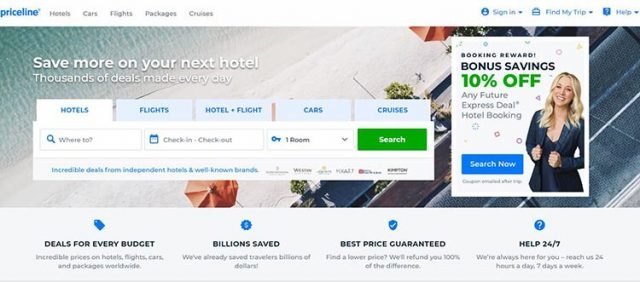The image is a desktop screenshot of the Priceline website, showcasing its extensive travel booking services. The top menu bar features options for booking hotels, cars, flights, packages, and cruises. In the upper right corner, there are links for "Sign In," "Find My Trip," and "Help."

The main section of the page prominently displays an aerial photograph of a picturesque beach. The top left corner of the photo features vibrant blue water, while a stretch of pristine white sand cuts diagonally across the middle. In the lower right-hand corner, part of a hotel's roof is visible. A headline reads, "Save more on your next hotel, thousands of deals made every day."

Directly below this headline are options for booking accommodations and travel: hotels, flights, hotel and flight packages, cars, and cruises. A search box offers input fields labeled "Where to?" along with a calendar for selecting check-in and check-out dates. A key symbol indicates the selection of "one room," with a drop-down menu for additional choices. The search process begins with a prominent green "Search" button.

On the right side of the page, there is a pop-up banner promoting "Bonus Savings" with a 10% discount on any future express deal hotel bookings. This banner features an image of a smiling, dyed blonde, white woman wearing a cardigan. The promotion can be accessed via the blue "Search Now" button.

Lastly, the bottom of the screen provides additional navigation options, enhancing the user’s ability to explore further booking and travel planning services.